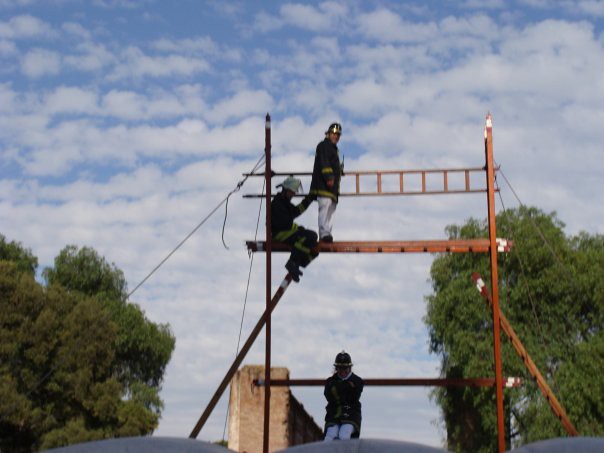The image depicts three firefighters involved in what appears to be a training or demonstration exercise on a makeshift scaffolding constructed from multiple ladders. The structure, which might resemble a staging area, is held in place by visible tie-downs and seems precariously high, with several ladders (potentially up to seven) forming its main framework. 

In the scene, two firefighters are positioned atop the scaffolding: one, wearing a white fireman’s hat along with regular jeans, is standing and facing towards the camera, seemingly holding a walkie-talkie. Another firefighter, wearing a dark-colored hat, is seated on the topmost ladder. A third firefighter, also in fireman's gear with lighter-colored pants, is positioned on the ground beneath the scaffolding, facing the camera but looking slightly downward.

The background features trees on both the left and right with a partly cloudy blue sky. Below the scaffolding's base, there appears to be a small brick or stone wall, and at the very bottom of the picture, three indistinguishable gray humps are visible. A ladder is hanging in front of the standing firefighter, potentially serving as a rail, and additional ladders can also be seen extending below the setup, contributing to the intricate appearance of the scene.